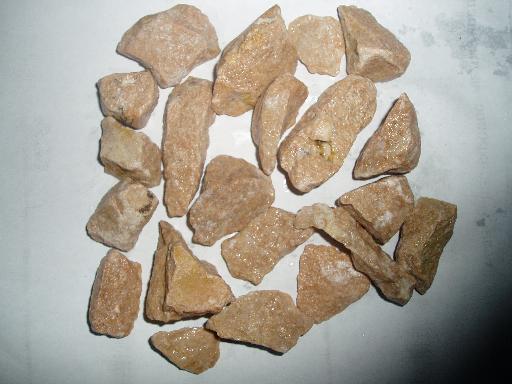The image depicts a collection of 21 light brown stones with hints of white, beige, and subtle pinkish-orange hues. The stones exhibit a lustrous sheen, possibly speckled with gold-like glitter, and vary significantly in shape and size. Some stones are tiny and rounded, while others are long, oblong, triangular, or square, with a few appearing sharply cleaved. They are arranged on a white surface that appears to have some smudges and features a black area in the lower right corner. The stones, resembling landscaping stones from a bag at a hardware store, are scattered in the center of the image, showcasing their diversity in form and texture.